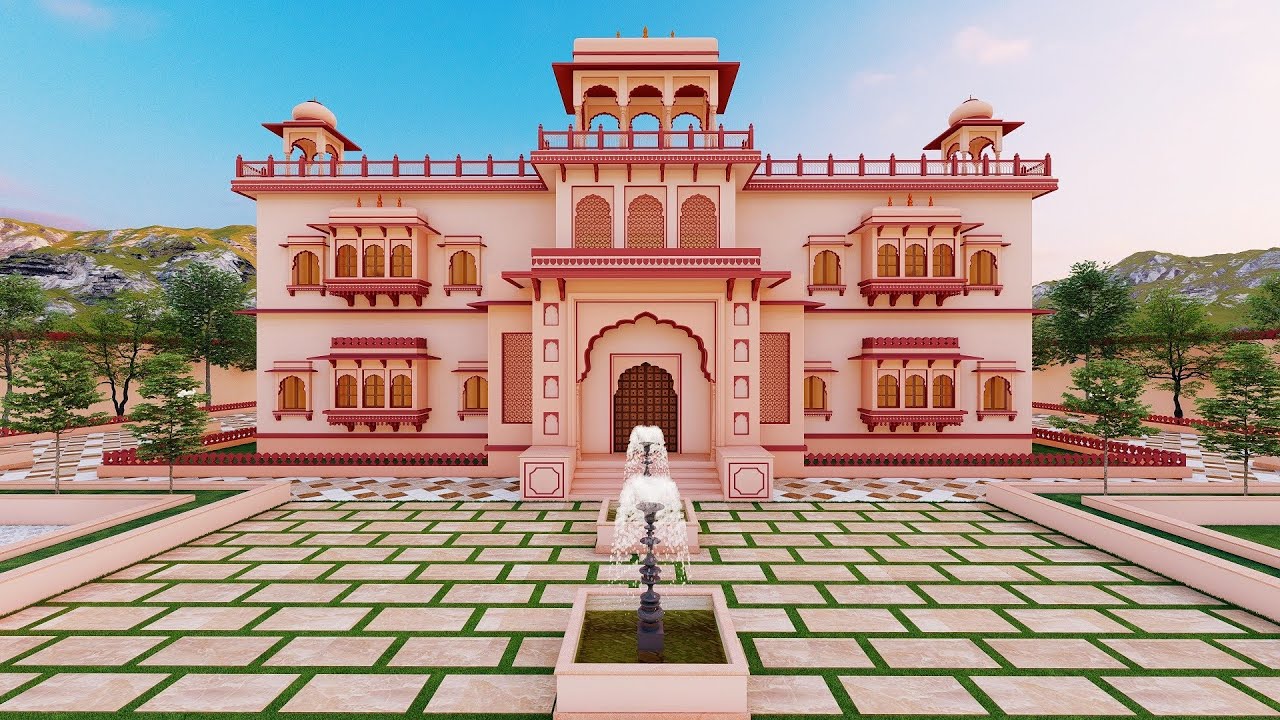The image depicts a symmetrical two-story villa with a blend of Moroccan and Indian architectural influences, characterized by its pinkish-red stucco exterior. The ornate building features numerous small windows and a flat rooftop bordered by a red railing, with three pavilions adorning the top. Below, there's an intricately designed courtyard paved with green stone paths interspersed with moss, extending fully around the villa. A sequence of square-shaped fountains, one in front of the other, punctuates the front courtyard, adding to the elegance. The overall setting is meticulously clean and well-maintained, complemented by a backdrop of softly rolling hills and mountains, partially covered in greenery and white splotches, under a bright blue sky that fades to white in the upper right corner. The landscape includes a walkway and channels filled with greenery, enhancing the sophisticated and serene ambiance of the scene.